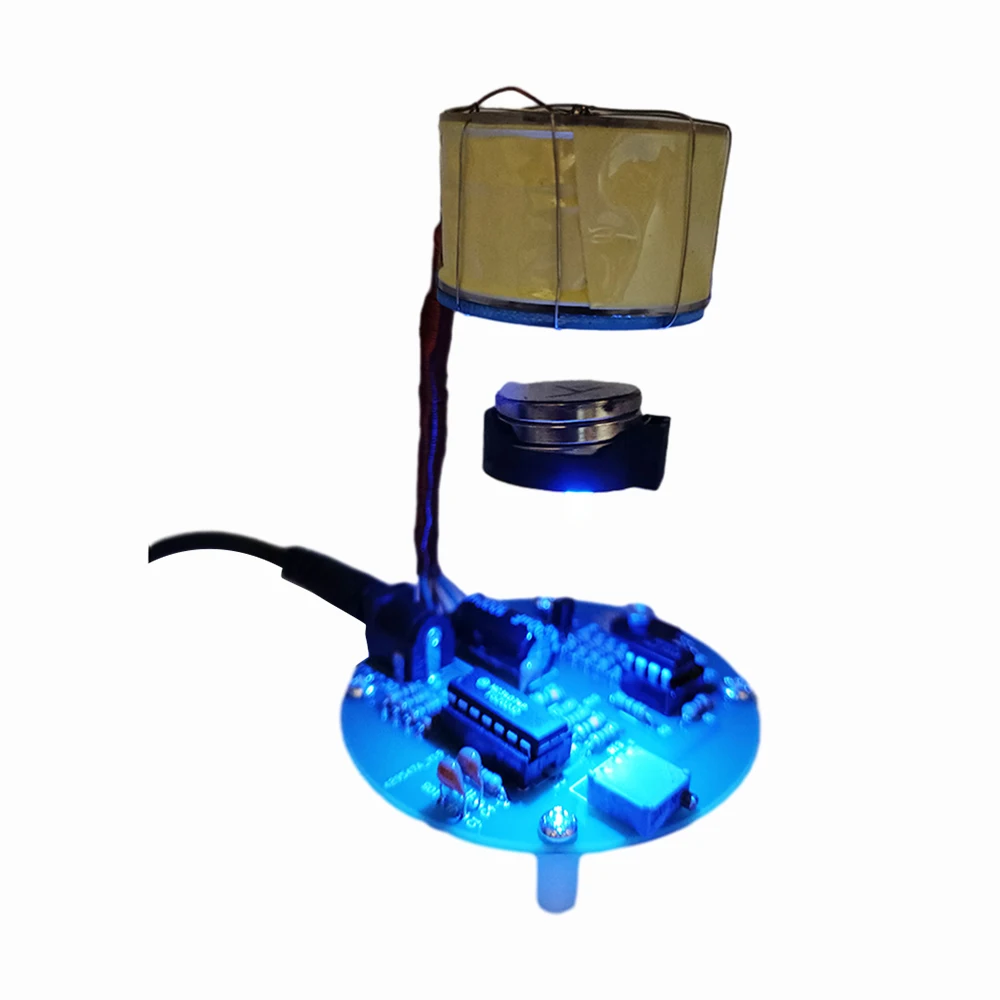This photograph features a detailed depiction of a mechanical device positioned against a white background. At the top of the device, a cylindrical, drum-like structure resembling a yellow lampshade is affixed. This lampshade-like top has a wire extending from it, which connects to the rest of the apparatus. Below this, a coiled metal component is visible within a round silver enclosure resting on a black base.

The lower section of the device comprises a circular disc, possibly made of a blue plexiglass-like material, which has various computer parts mounted on it, including small transformers, resistors, and what appears to be a small battery area. Blue light emanates from this disc, illuminating the surrounding components. A cord also extends from the back of the disc. Overall, the device showcases a combination of mechanical and electronic elements merged into a cohesive unit, suggesting it might serve as a functional light or experimental gadget.